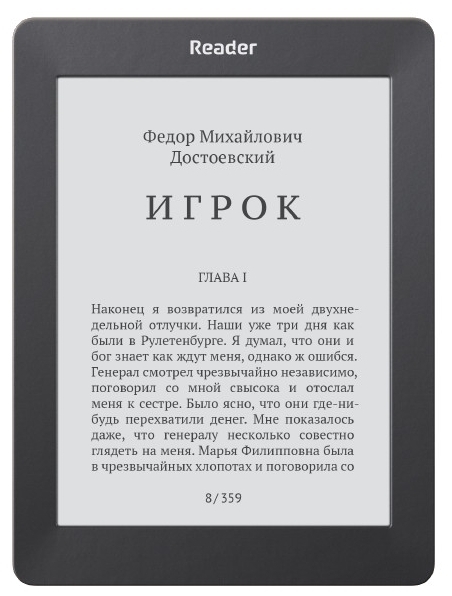The image showcases a Kindle reader with a large black frame and a gray background. At the top of the device, the word "Reader" is prominently displayed in white text. The screen itself features text in what appears to be Russian, displayed against a typical white background with black letters. At the top of the text, there's an indication of "chapter," followed by five larger letters, a space, and smaller letters below, likely part of a chapter heading. Beneath this, the main content appears as a paragraph. The bottom of the screen indicates the page number, 8 of 359, suggesting this is a digital version of a lengthy text.